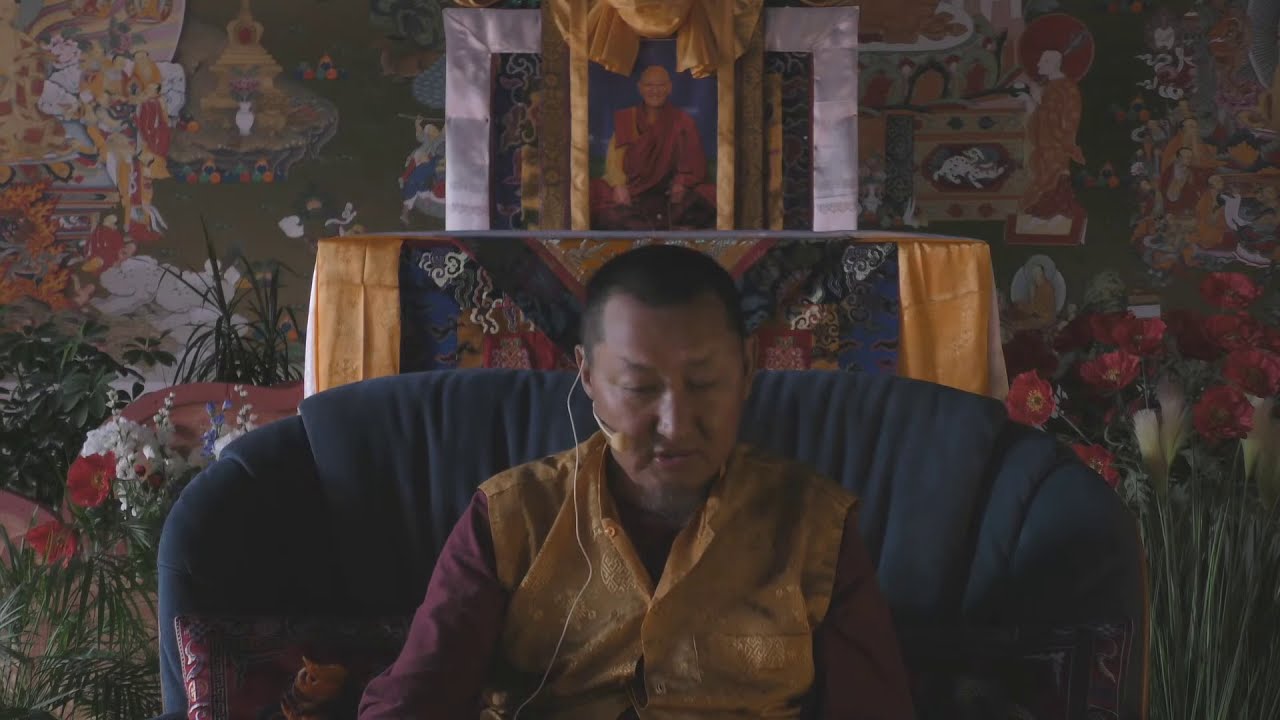The image features an Asian man, possibly Indian, seated in a large, dark-colored chair, described variably as black, dark green, or navy blue. He is dressed in a glittering yellow-orange shirt with maroon or red sleeves. The man is wearing a white microphone headset with a wire visible on his left side and appears to be looking down, potentially engaged in a conversation or call.

Behind him, there's an elaborately framed photograph of another monk adorned in red and orange robes with a gold emblem on top, suggesting a shrine or significant display. This backdrop includes intricate designs, resembling busy wallpaper featuring trees, leaves, and flowers in browns, golds, and reds. Additionally, there are red flowers with green stems flanking the central photograph, enhancing the spiritual or ceremonial ambiance of the scene.